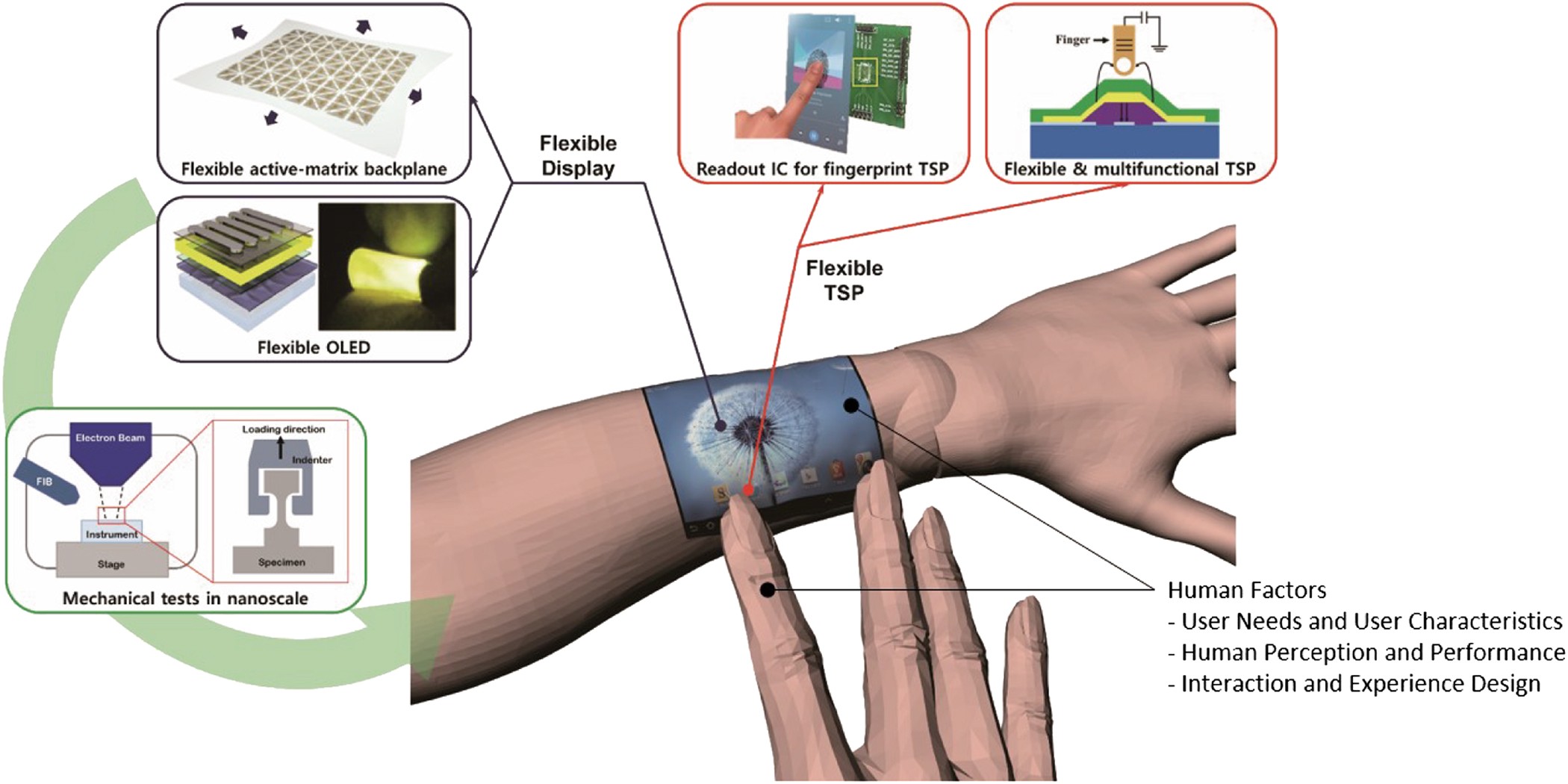The image is a horizontally rectangular, multi-color, computer-generated illustration set against a plain white background. At the center, there is a prominent depiction of a forearm with an extended hand and four fingers. Attached to the wrist is a blue device labeled "Flexible TSP," which features a graphic resembling a dead dandelion's white ball. Text around the image lists various technological and user-centric terms, including "Flexible Active Matrix Backplane," "Flexible OLED," "Flexible Display," "Readout IC for Fingerprint TSP," "Flexible and Multifunctional TSP," and "Human Factors, User Needs and User Characteristics," as well as "Human Perception and Performance, Interaction and Experience Design," and "Mechanical Tests in Nano Scale." This suggests that the image represents a conceptual wrist-mounted computer device integrating flexible display technology and advanced user interface considerations.